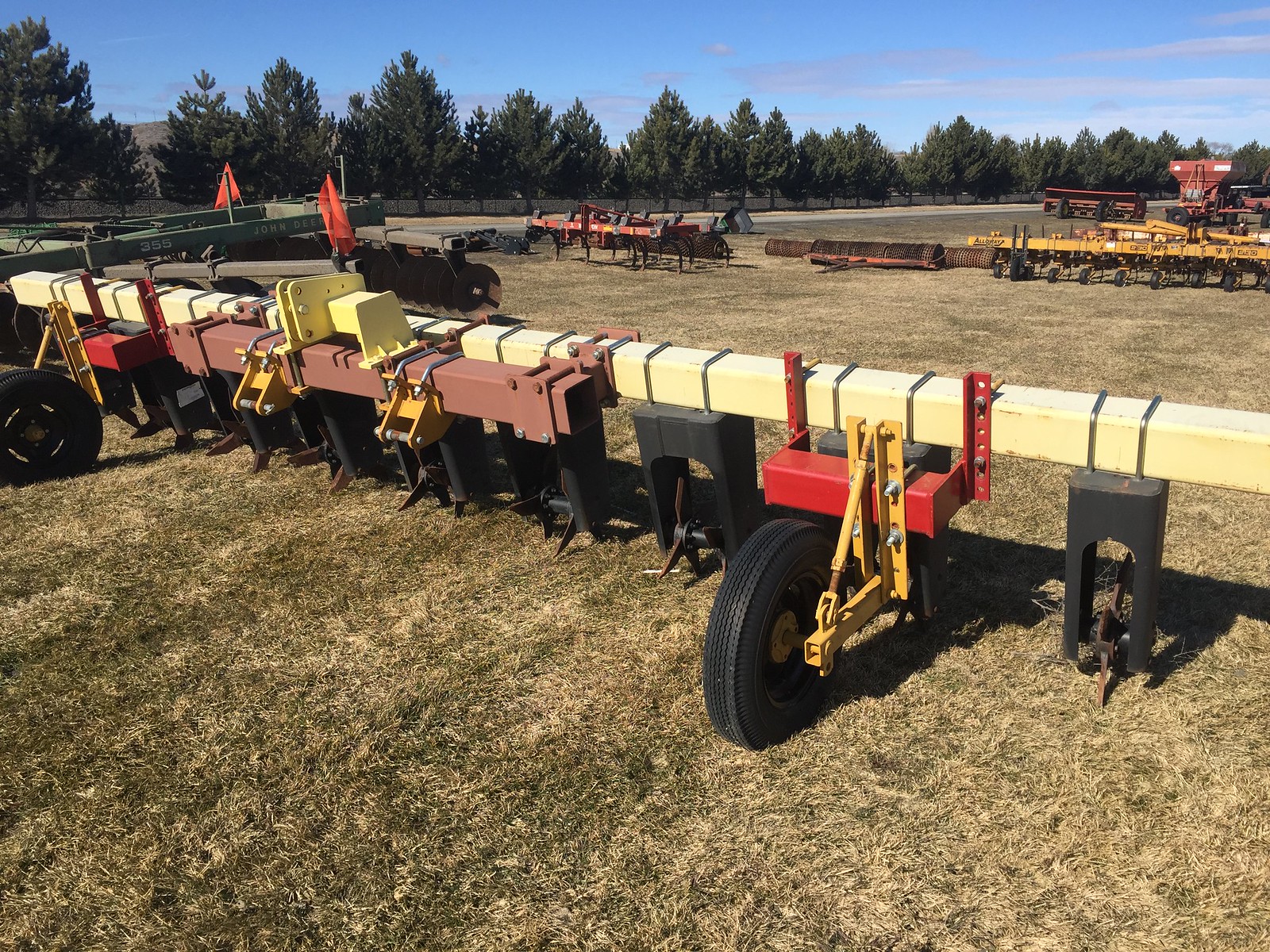In this vibrant outdoor photograph taken on a sunny day, the scene is set with natural lighting that highlights a large expanse of pastureland. The field in the foreground is predominantly yellowish-brown, indicating dry conditions, interspersed with patches of green grass. Critical to the image is a long, narrow piece of farming equipment extending at an angle from the center-right to the upper-left. This machinery features a yellow beam with red brackets holding its wheels, which are equipped with yellow hydraulic mechanisms designed to adapt to the field's uneven terrain. Surrounding the field, the background boasts a line of dark green, likely evergreen trees, creating a natural frame for the scene. Above these trees, the sky is bright blue with a few thin white clouds, adding to the sunny ambiance. The distant background also includes what appears to be additional farming apparatus, highlighting the agricultural setting of this expansive landscape.